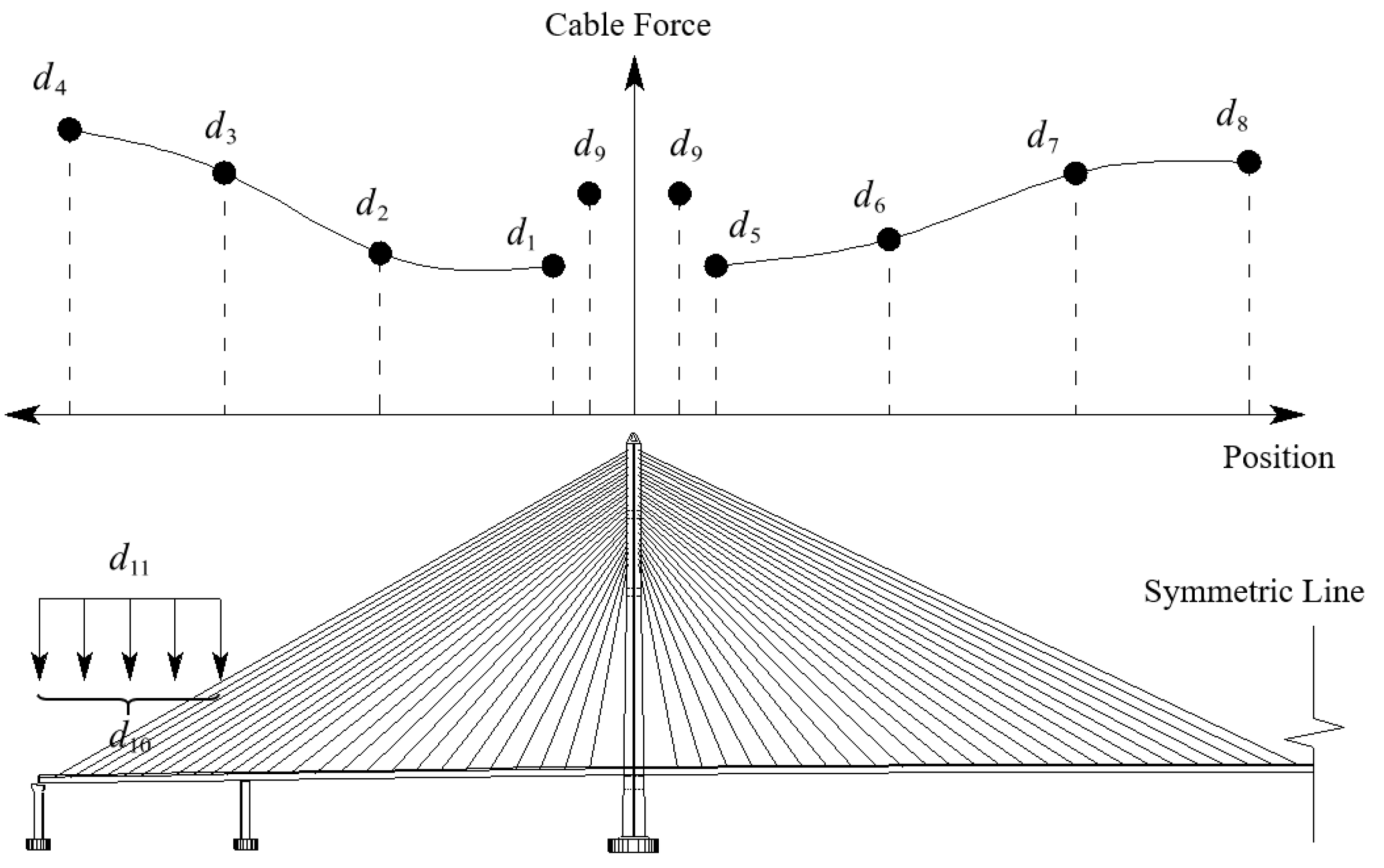The image is a detailed engineering diagram, likely related to physics, illustrating the structure and function of a suspension bridge. The diagram features a long horizontal line representing the bridge road, supported by a vertical structure in the center. Multiple cables of varying lengths extend from this central structure, creating a lattice-like appearance that resembles harp strings. These cables are labeled with a sequence of designations such as D1, D2, D3, up to D9, marking their different positions and lengths. At the top of the diagram, the term "cable force" is prominently displayed, with accompanying arrows that point in different directions, indicating the forces exerted by the cables to support the bridge. Additionally, there's a line of symmetry highlighted by the label "symmetric line," suggesting the equal distribution of these forces across the structure. Equations and mathematical notations are scattered across the diagram, further emphasizing its technical and analytical nature.